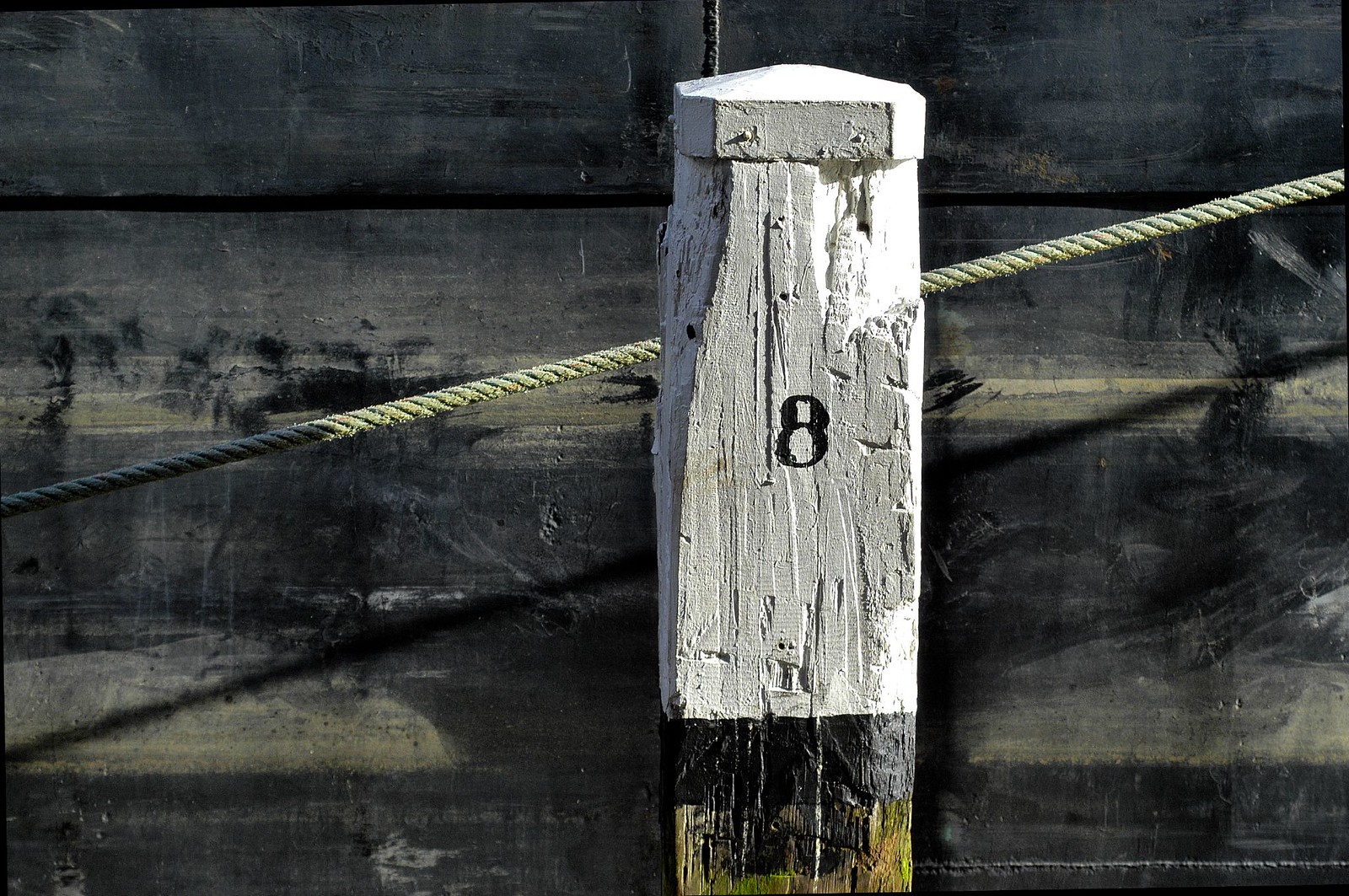This photograph captures a very weathered and beaten wooden post set against a rough, grayish-brown wooden backdrop. The post, painted white at the top, prominently features a black number 8 in the middle section. Below the number, the post is marked with thinner black paint and transitions into its natural weathered wood appearance, showing brown hues with green patches from algae or moss. The bottom portion of the post displays significant wear, exposing black and possibly yellow highlights. Diagonally through or behind the post, there are two taut strands of manila rope, suggesting a setting akin to a pier. The sun illuminates the post and rope, casting subtle shadows, while the background wall appears to consist of weathered slapboard planks in shades of gray and dark gray.